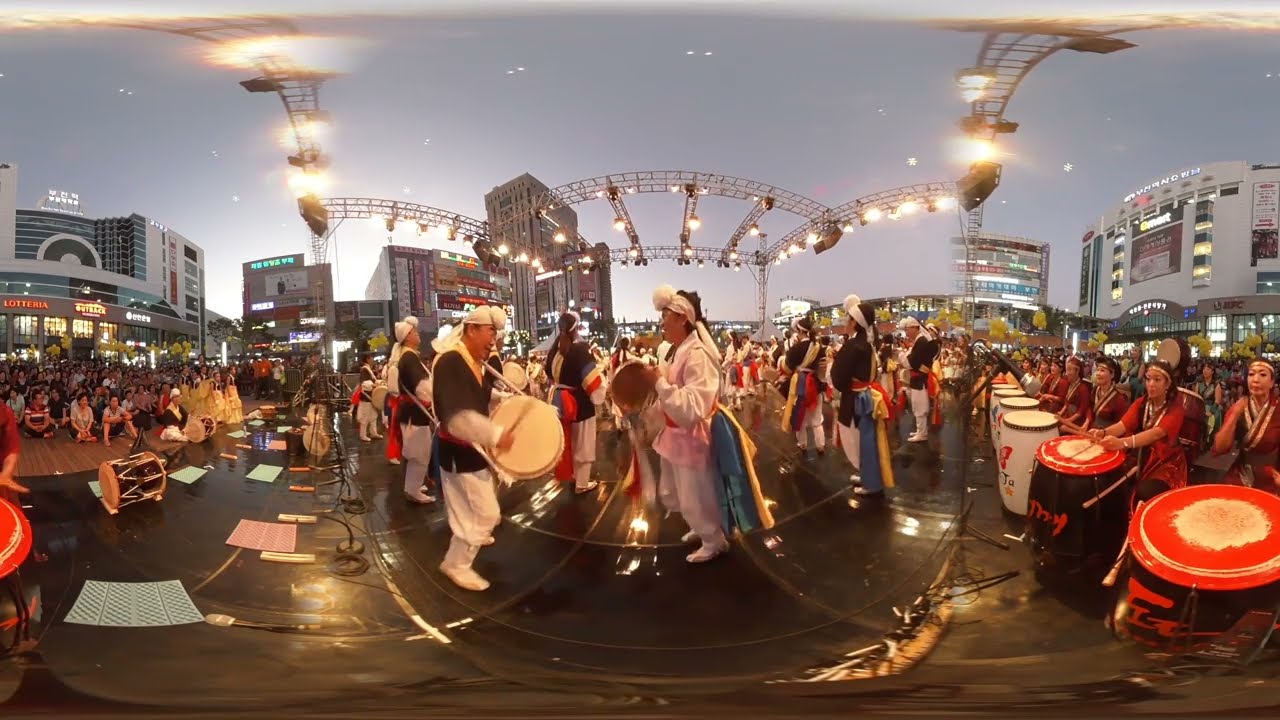The image captures a lively street festival or performance set within an urban landscape at dusk. Central to the scene are two men facing each other, deeply engaged in drumming. One man is dressed in a black shirt and white pants, playing a white drum with white detailing on his sleeve. His counterpart, clad entirely in white with a red sash around his waist and a white rag wrapped around his face, adds a striking contrast. Above them, there is scaffolding adorned with orange lights, suggesting the top of a stage setup. The ground beneath them is a shiny black surface, dotted with vents in pink and light blue colors, reflecting the overhead lighting.

To the far right, a line of drums—starting with black and white ones, followed by red ones—are manned by women in red costumes, some actively playing. The street curves from the left, forming a circular pattern as it traverses the scene. Surrounding the central performance area, an audience seated on the ground implies an immersive and inclusive atmosphere. In the background, tall buildings with modern architecture dominate, including a light gray building with blue glass windows on the left and another gray building on the right with bright, illuminated signage. The sky, painted in shades of gray and blue with scattered white dots, encapsulates the image in the dim light characteristic of dusk.